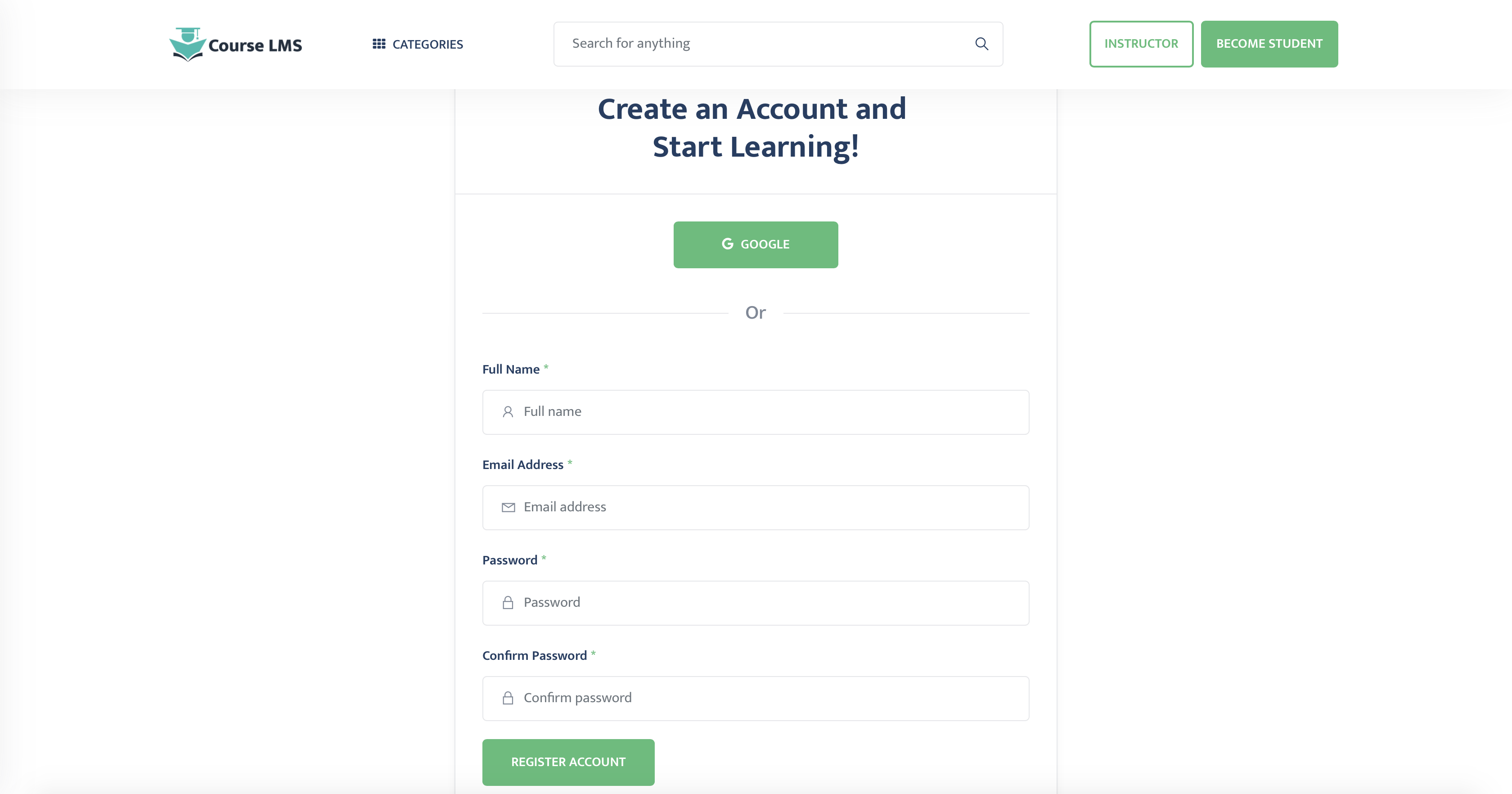This screenshot features an interface from an online learning website branded as "Course LMS." In the upper left-hand corner, the "Course LMS" logo prominently identifies the platform. Directly to the right, a category submenu allows for easy navigation through various course topics. Adjacent to the submenu, a search bar is available for users to find specific courses or content on the website.

Further along the top navigation bar are two buttons: "Instructor Login" and "Become Student Login," facilitating access for both educators and learners. 

The main section of the window contains a welcoming call-to-action message: "Create an account and start learning." Users are given two options to create an account: they can either sign in using their Google account for a quicker registration or manually enter their name, email address, and a password to set up a new account from scratch. This clearly structured interface aims to make the process of joining and participating in courses straightforward and user-friendly.